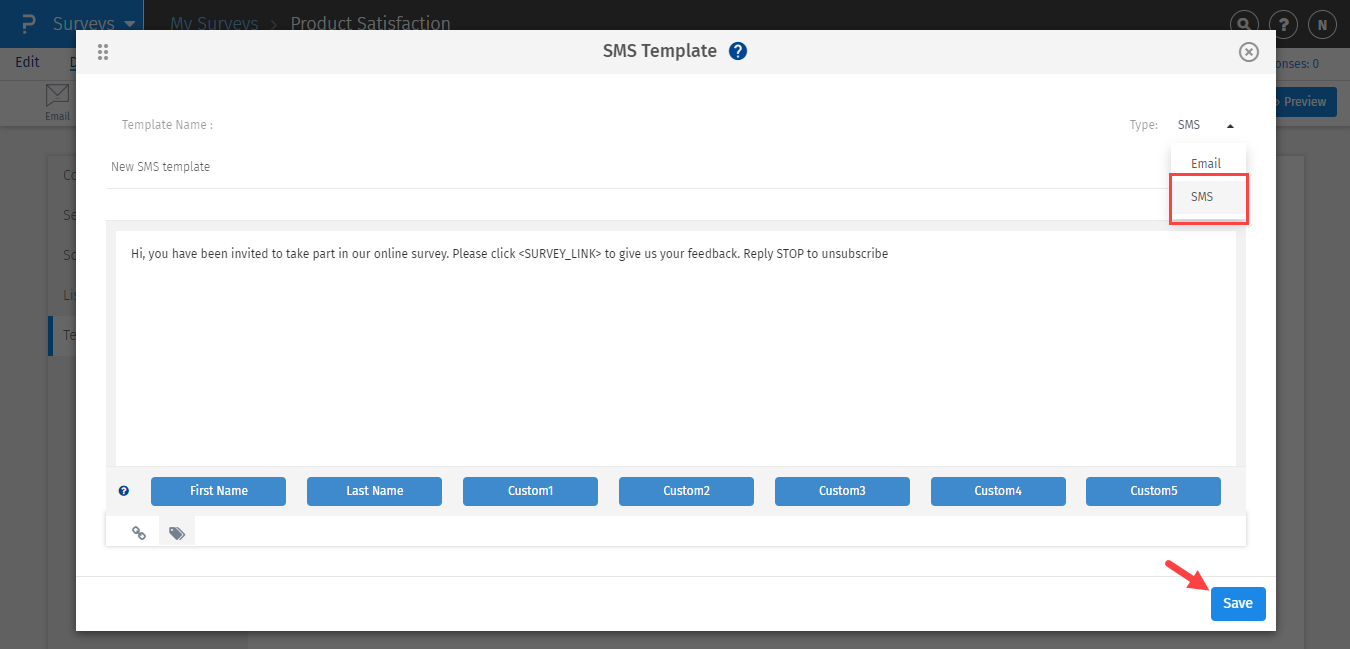This is a screenshot captured from an unidentified online platform. The image prominently features a white pop-up window titled "SMS Template" overlaying the main web page. Inside this window, there is a large text area containing the following message: "Hi, you have been invited to take part in our online survey. Please click [survey link] to give us your feedback. Reply STOP to unsubscribe." Below the text area are seven rectangular blue buttons, the exact labels of which are not legible. At the very bottom of the window, a blue "Save" button is clearly visible, suggesting that the user can save the new SMS template after making any changes.